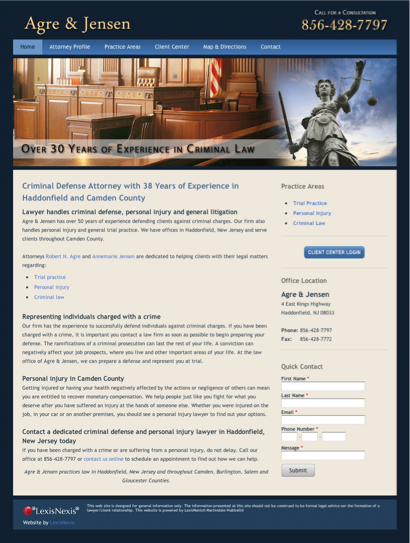**Website Banner for AGRE & Jensen Criminal Lawyers**

The webpage for AGRE & Jensen Criminal Lawyers features a professional banner designed to convey trust and expertise. At the top, a navigation menu includes tabs such as Home, Attorney Profiles, Practice Areas, and a Client Center Login button. 

The banner prominently displays an elegant statue of the scales of justice, symbolizing fairness and balance, alongside an image of a courtroom that underscores their legal focus. An impressive banner text proclaims “Over 30 Years of Expert Experience in Criminal Law,” reflecting the firm’s longstanding service.

Highlighted in blue at the bottom of the image is the firm’s contact number, 856-428-7797, and a brief introduction: “A criminal defense attorney with 38 years of experience in Haddonfield and Camden County.” The text outlines the practice areas including Criminal Defense, Personal Injury, and General Litigation, further detailing their expertise in Trial Practice and Criminal Law.

A section beneath emphasizes their mission: “Representing individuals charged with a crime and personal injury in Camden County. Contact a dedicated criminal defense and personal injury lawyer in Haddonfield, New Jersey, today.”

Completing the webpage banner is a contact form for quick inquiries, featuring fields for First Name, Last Name, Email, Phone Number, Message, and a convenient Submit button. The firm's office location is specified, ensuring potential clients can easily reach out.

This detailed and informative banner sets a professional tone for the services offered by AGRE & Jensen, promising dedicated legal support for individuals in need.